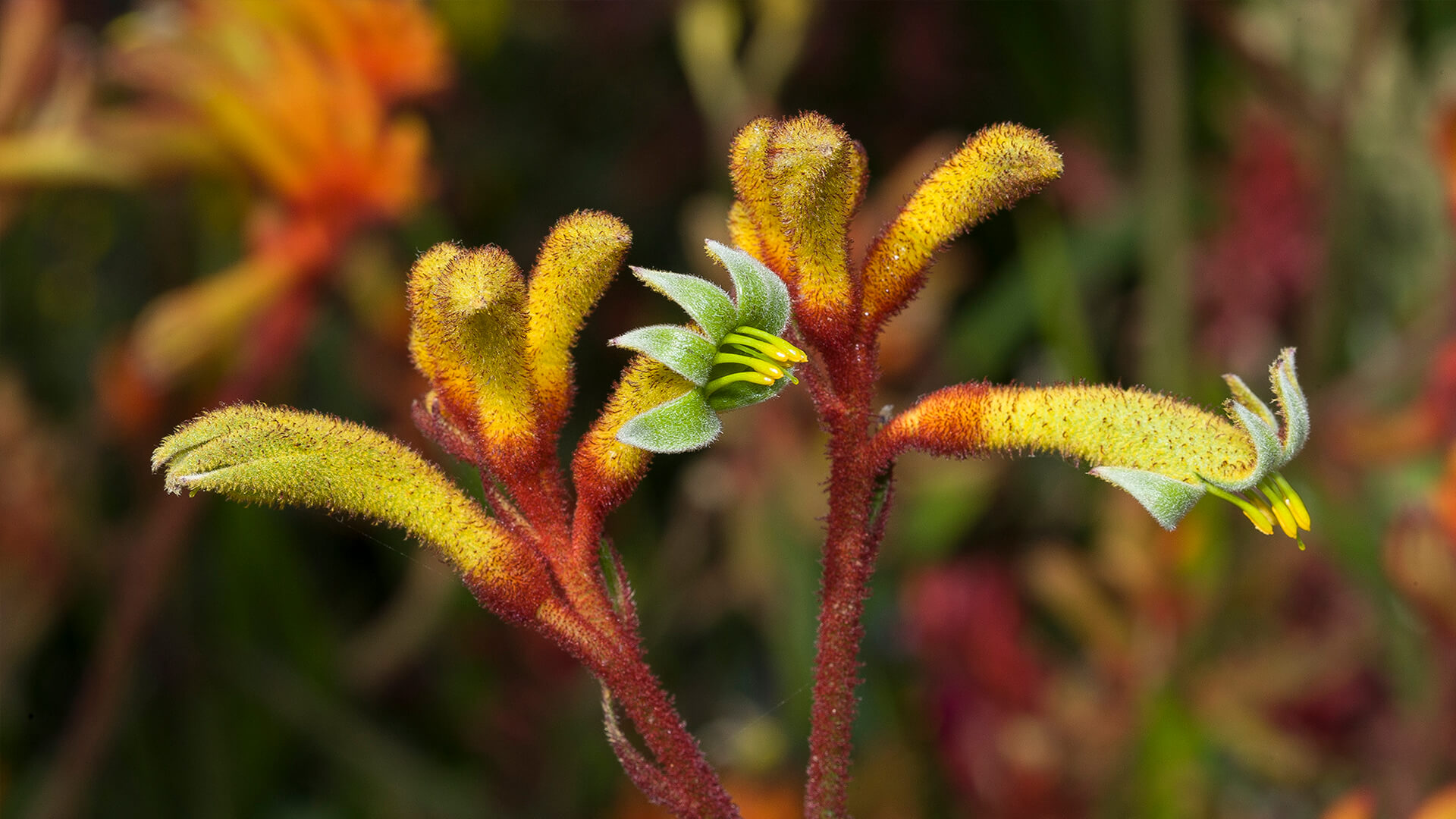This detailed image captures an up-close shot of a vibrant flower in transition. The deep red stems, adorned with fine red hairs, ascend to the top where they transform into narrow yellow-green blooms. Some of the flowers are just beginning to open, revealing layers of yellow petals and possibly emitting pollens. Emanating from the center, the stems radiate a carpet of fuzz, giving the entire structure a soft, fur-covered appearance. In the background, a blurred array of similar flowers and abundant plant life create a vivid tapestry of greens, reds, yellows, oranges, and burgundies. The interplay of sharp detail and soft focus enhances the complexity and beauty of the flowering plant, accentuating its striking colors and unique textures.